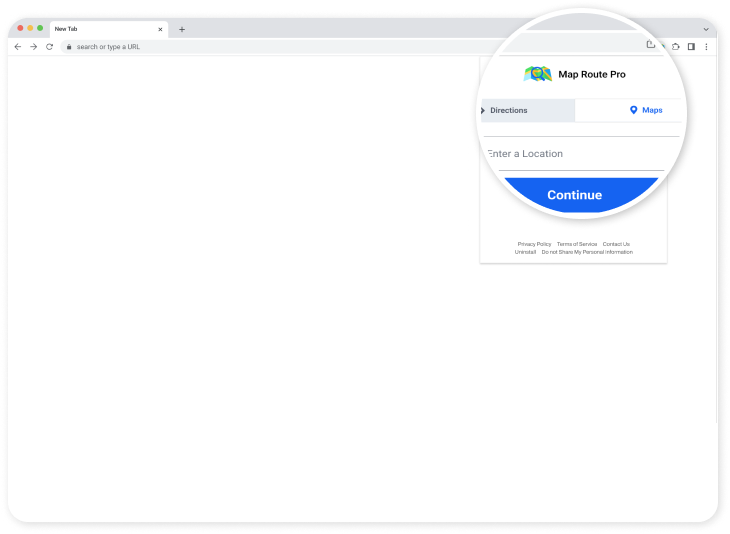The image depicts a new tab interface, presumably on an Apple device, as indicated by the red, yellow, and green dots in the upper left corner typical of macOS windows. The central area features a prominent, oval-shaped search bar with the prompt "Search or type URL." 

In the upper right-hand corner, a magnified section shows options for "MapRoot" and "ProSearch" with directions to access maps. Below these options is a blue "Continue" button with white text. Additional links under the button include "Privacy Policy," "Terms of Service," "Contacts Uninstalled," and "Do Not Share My Personal Information."

The upper right section of the interface contains options for accessing Gmail, a personal profile, a settings menu, and another unidentified feature. The rest of the page is blank, suggesting it may not have fully loaded or is a placeholder page. The absence of any Google branding, despite similarities to Google's typical layout, indicates an incomplete or partially loaded state.